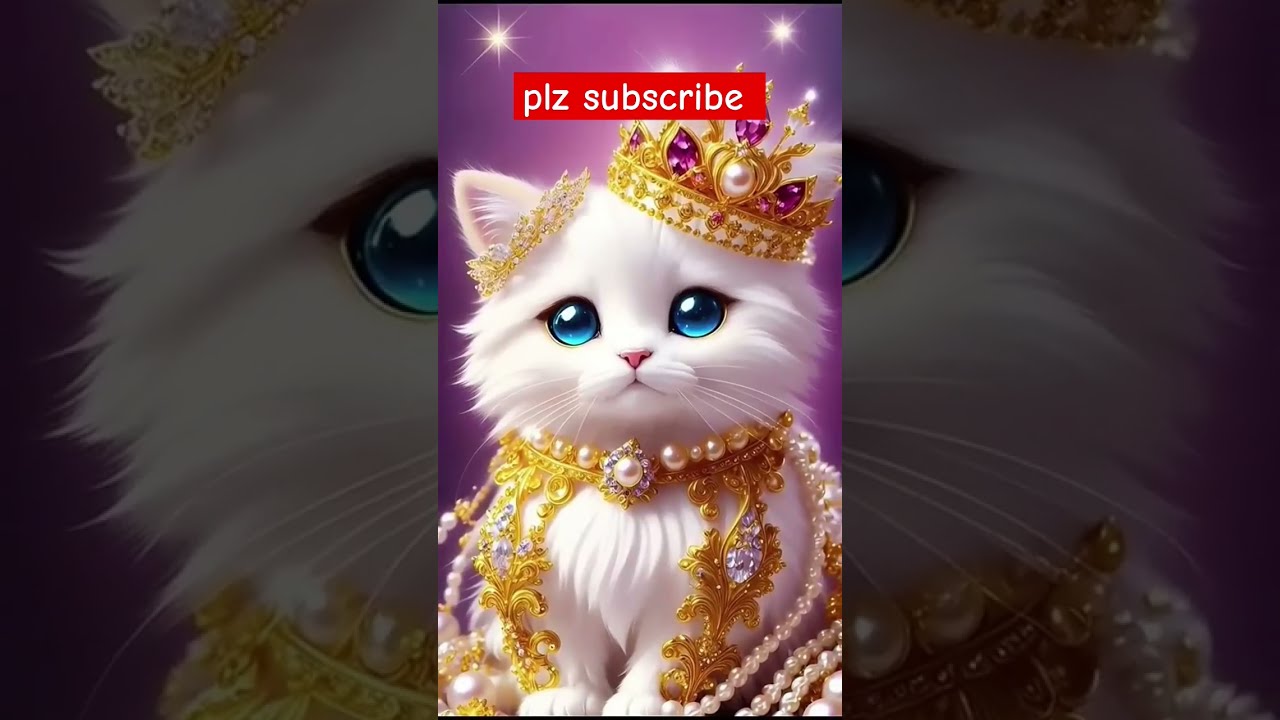This horizontal rectangular image, likely a screenshot from a video game or digital advertisement, features a central vertical rectangle displaying a striking white kitten adorned in opulent regalia. The kitten, positioned centrally in the image, gazes directly at the viewer with large, expressive blue eyes that are accented with black eyeliner. It has a soft pink nose and white whiskers, enhancing its endearing appearance.

Around its neck, the kitten wears an elaborate necklace comprised of gold with a leaf pattern, interspersed with pearls and diamond accents, and cascading chains of pearls down its sides. Additionally, a gold crown rests diagonally over its ear, adorned with violet-colored rubies, a prominent white pearl in the center, and surrounded by diamonds.

The background of the image is predominantly purple with sparkly white stars dotted across the top, giving a celestial feel. Above the kitten's head, against a red rectangular background, bold white letters read "PLZ subscribe." Flanking the central image on either side are darker, close-up vertical rectangles highlighting each side of the kitten's face. The overall color palette includes purple, white, red, tan, gray, silver, and gold, contributing to the image's rich, fantastical theme.